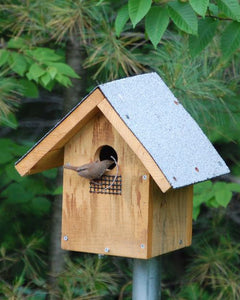This image captures a wooden birdhouse perched on a silver metal pole amidst lush green leaves and plant needles. The birdhouse is constructed from unfinished light brown wood and capped with a light gray roof, possibly made of tar or metal, which adds a waterproof layer. At the front of the birdhouse, a small bird, perched on a grid under the entrance hole, is seen with its body outside and its head peering into the hole. In its beak, the bird carries a twig, likely for nest building, suggesting it is in the process of creating a home within the birdhouse. The surroundings of dense greenery enhance the simplicity and natural placement of the birdhouse, typical of suburban settings, designed to deter squirrels and larger birds from invading the nesting space.